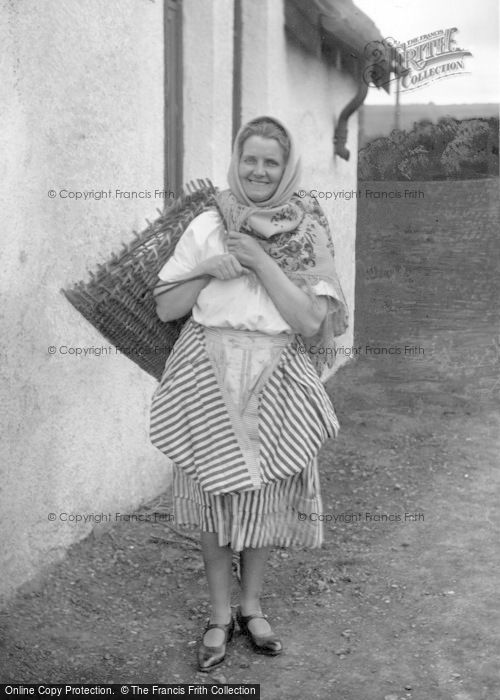The black and white image features a middle-aged woman standing on a dirt path next to a stone building, which is slightly to her left. The woman is dressed in basic, old-fashioned clothing reminiscent of farmhand attire, including a raggedy dress or skirt that appears puffy and oddly folded at the front, and a shawl draped over her head and shoulders. She carries a hay basket slung over her right shoulder. The landscape in the background consists of some bushes and generally open, empty fields, suggesting a rural setting. The composition feels historical, possibly dating back to the 1930s or 1940s, indicative of a poorer country. There's a noticeable watermark and text throughout the image reading "Online Copy Protection, The Frances Frith Collection, Copyright Frances Frith" with a logo at the top right and multiple watermarks dispersed across the photo. The woman, who appears white and is wearing dress shoes incongruously for farm work, is centered in the image, and she's smiling slightly under a cloudy, daylight sky.